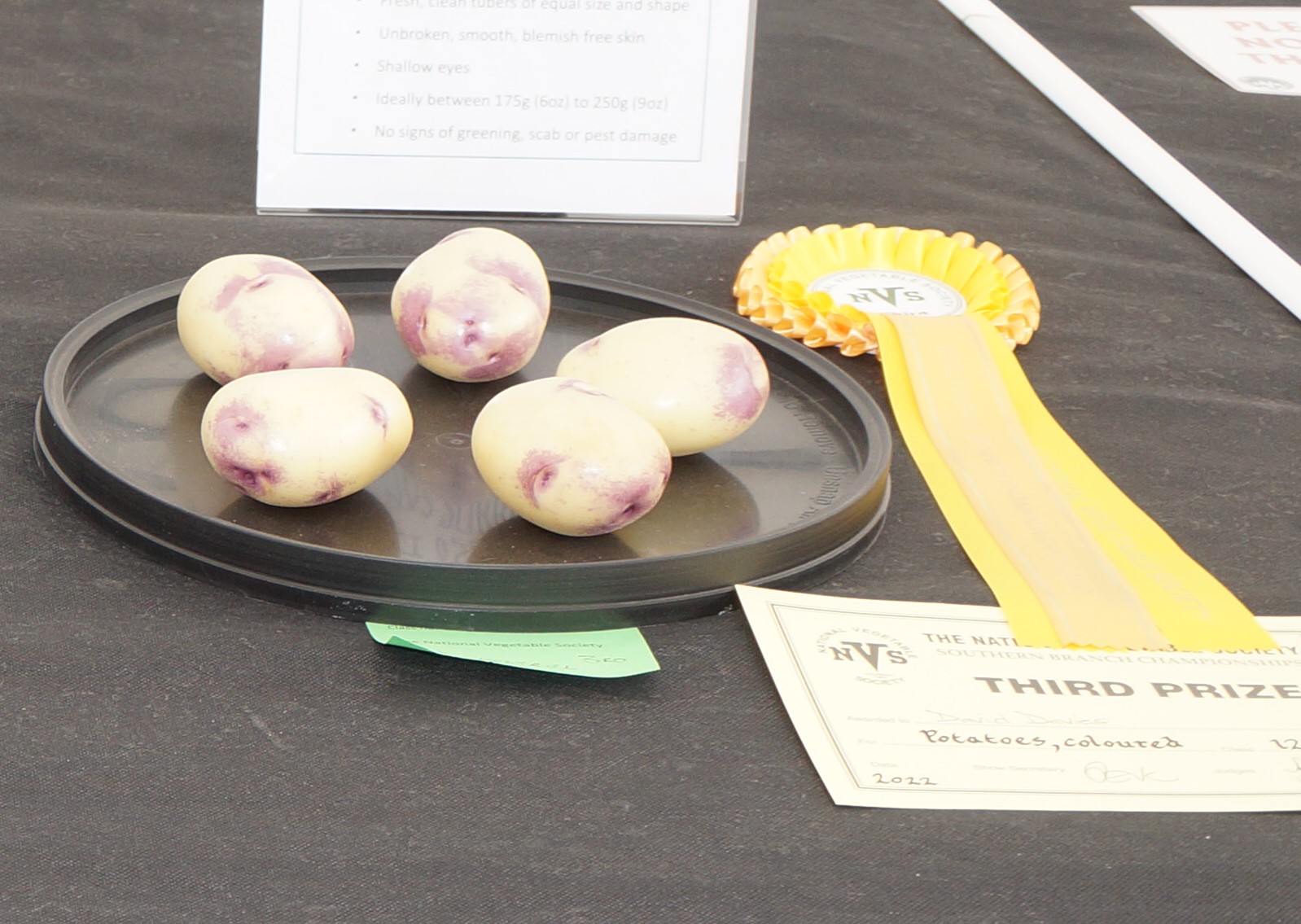The image depicts a display at what appears to be a county fair or a similar contest setting. Centered on a table with a black cloth is a black plastic plate containing five uniquely attractive potatoes. These potatoes, which are white with bluish-purple splotches, are meticulously arranged in a star-like formation. They have been awarded third prize, indicated by a prominent yellow rosette beside them and a certificate that reads, "Third Prize, Potatoes, Colored." Behind the plate, partly obscured, is a detailed sign outlining the criteria for prize-winning potatoes. The criteria include having fresh, clean tubers of equal size and shape, unbroken and smooth skin, shallow eyes, ideally weighing between 175 grams to 250 grams, and showing no signs of greening, scab, or pest damage. The sponsoring organization, NVS, is also mentioned in the certificate.